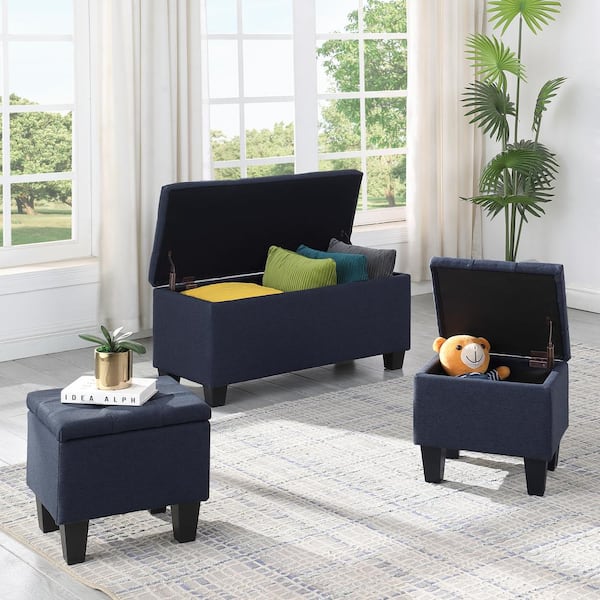The image showcases a simple, minimalistic room with floor-to-ceiling windows that have white panes and plain white curtains, allowing a clear view of a lush green landscape with trees and grass outside. Inside the room, three pieces of navy blue storage furniture are arranged in a triangle formation: two small ottomans at the front and a larger chest-like piece at the back. The left ottoman is closed, topped with a white book titled "Idea Elf" and a brass pot containing a small green plant, possibly a succulent. The right ottoman is open at a 45-degree angle, revealing a small teddy bear inside. The larger chest at the back is also open, containing four throw pillows in yellow, green, teal, and gray. A tall, green palm-fronded plant sits in the back corner of the room. The floor appears to be tiled, contributing to the room's clean, minimalistic aesthetic.